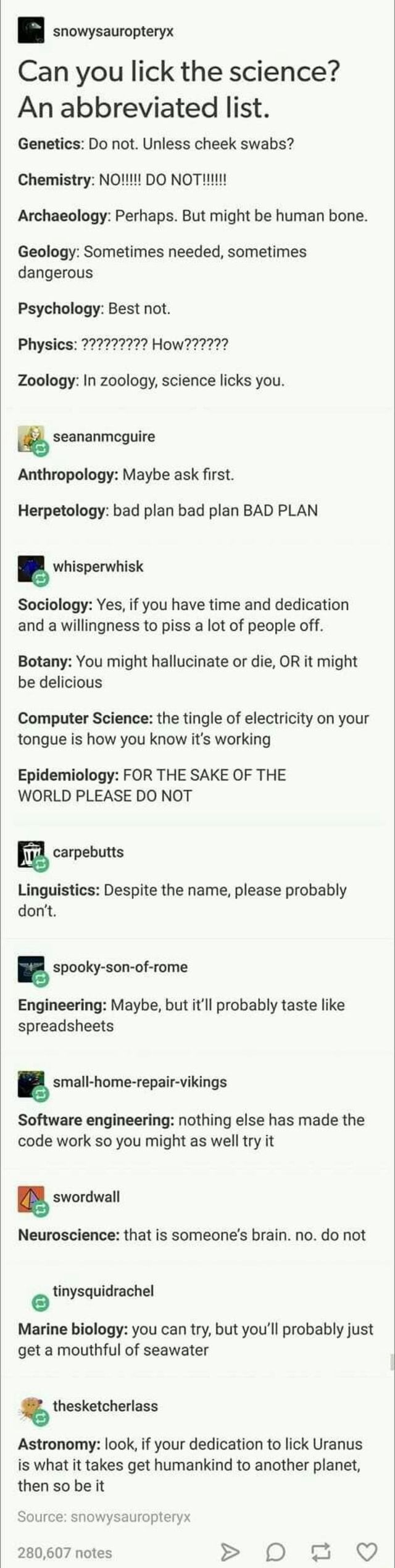Here is the detailed and cleaned-up description for the image caption:

---

The image features a humorous and detailed conversation thread on a social media wall, the background being a subtle off-white, with all text written in black. The conversation appears to revolve around different scientific disciplines and the hypothetical, often comical consequences of "licking" various branches of science. At the top is the username "snowysauropteryx" who initiates the discussion with the prompt: "Lick the science?"

Below this prompt is an abbreviated list of sciences and the repercussions of licking them:
- Genetics: "Do not, unless cheek swabs?"
- Chemistry: "No, do not!!!"
- Archaeology: "Perhaps, but might be human bone?"
- Geology: "Sometimes needed, sometimes dangerous?"
- Psychology: "Best not."
- Physics: "How?"
- Zoology: "In zoology, science licks you."

Following “snowysauropteryx,” various other users contribute:
- Sean Ann McGuire (Sheenan McGuire): "Anthropology: maybe ossfass?" "Herpetology: bad plan, bad plan, bad plan."
- Whisperwhis: "Sociology: yes, if you have the time, dedication, willingness to piss off a lot of people." "Botany: You might hallucinate or die, or might be delicious." "Computer Science: The tingle of electricity on your tongue is how you know it's working." "Epidemiology: For the sake of the world, please do not."
- Carpebut: "Linguistics: Despite the name, please probably don't."
- Spooky Son of Rome: "Engineering: Maybe, but it'll probably taste like spreadsheets." "Small home repair Vikings: Software engineering, nothing else has made the code work, so you might as well try it."
- A Word War: "Neuroscience: That is so much brain, no, do not."
- Tiny Quadracle: "Marine Biology: You can try, but you'll probably just get a mouthful of seawater."
- The Sketchiless: "Astronomy: Look, if your dedication is to lick Uranus is what it takes to get humankind to another planet, then so be it."

The thread paints a vivid and amusing picture of the perils and peculiarities associated with each field if approached in the most literal sense.

---